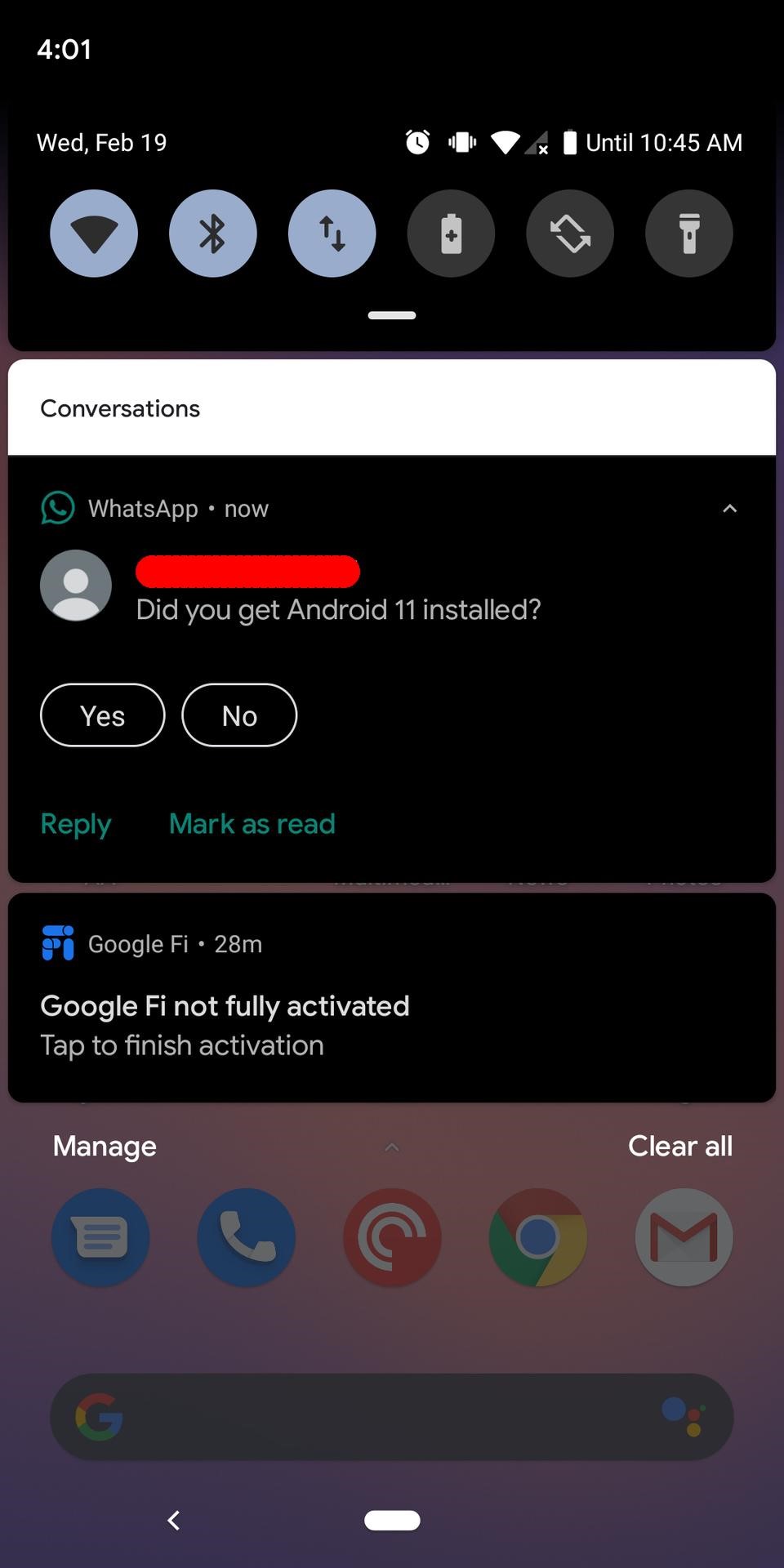The screenshot showcases a phone's lock screen at 4:01 AM on Wednesday, February 19. The device's background is a solid black, making the white text and icons pop. At the top, the current time is prominently displayed, followed by the date. An icon of an alarm clock or stopwatch appears next to the time information. 

A battery icon indicates that the battery is fully charged, with a text beside it reading "until 10:45 AM". Below the battery icon, there are two gray circles: one contains a battery icon, and the other a flashlight icon, both in light gray.

A white horizontal bar with the text "Conversations" in black separates the screen's elements. Beneath this bar, there is text indicating that the WhatsApp app is active. A green chat bubble with a white phone icon inside it is adjacent to this text.

Further down, a red line approximately one inch long appears, under which a message reads, "Did you get Android 11 installed?" in white text. Following this message are two ovals outlined in white, reading "Yes" and "No," respectively. 

At the bottom, two green options are available: "Reply" and "Mark as read." Additionally, there is a blue circle with a white phone icon inside it. The Google logo, a multicolored letter "G," is also visible.

This detailed description paints a clear picture of the phone's lock screen, highlighting the various icons, messages, and notifications present.